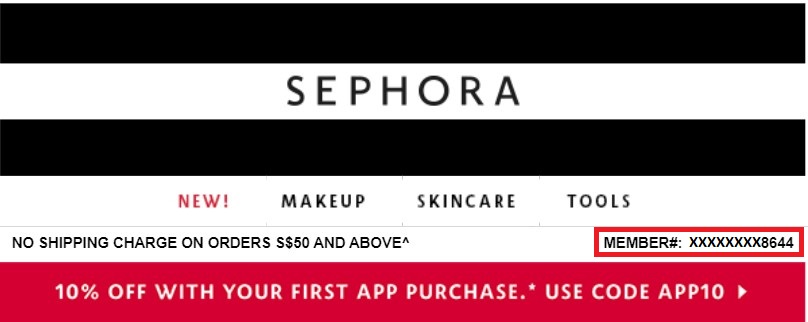This image showcases the header section of Sephora's website. The top section features a classic black navigation bar spanning the entire width. Directly below, there is a slim white bar with all capitalized letters in black providing navigation options. Under that, another black bar thrusts into focus. Following this, a wider white bar includes a red "NEW!" in capital letters, and subsequent categories like "MAKEUP," "SKINCARE," and "TOOLS," all in black text. Beneath these, the white bar continues, stating "No shipping charge on orders of $50 and above," albeit with a typo showing an extra 'S' before the dollar sign. There's also a section displaying "Member number" with a placeholder ending in 8644, highlighted in red. Another horizontal bar includes the promotion "10% off with your first app purchase. Use code APP10," featuring a right-pointing white arrow. The website's header ends at this point, offering no product details or clickable links, serving solely as an introductory display of Sephora's distinctive black and white brand style.